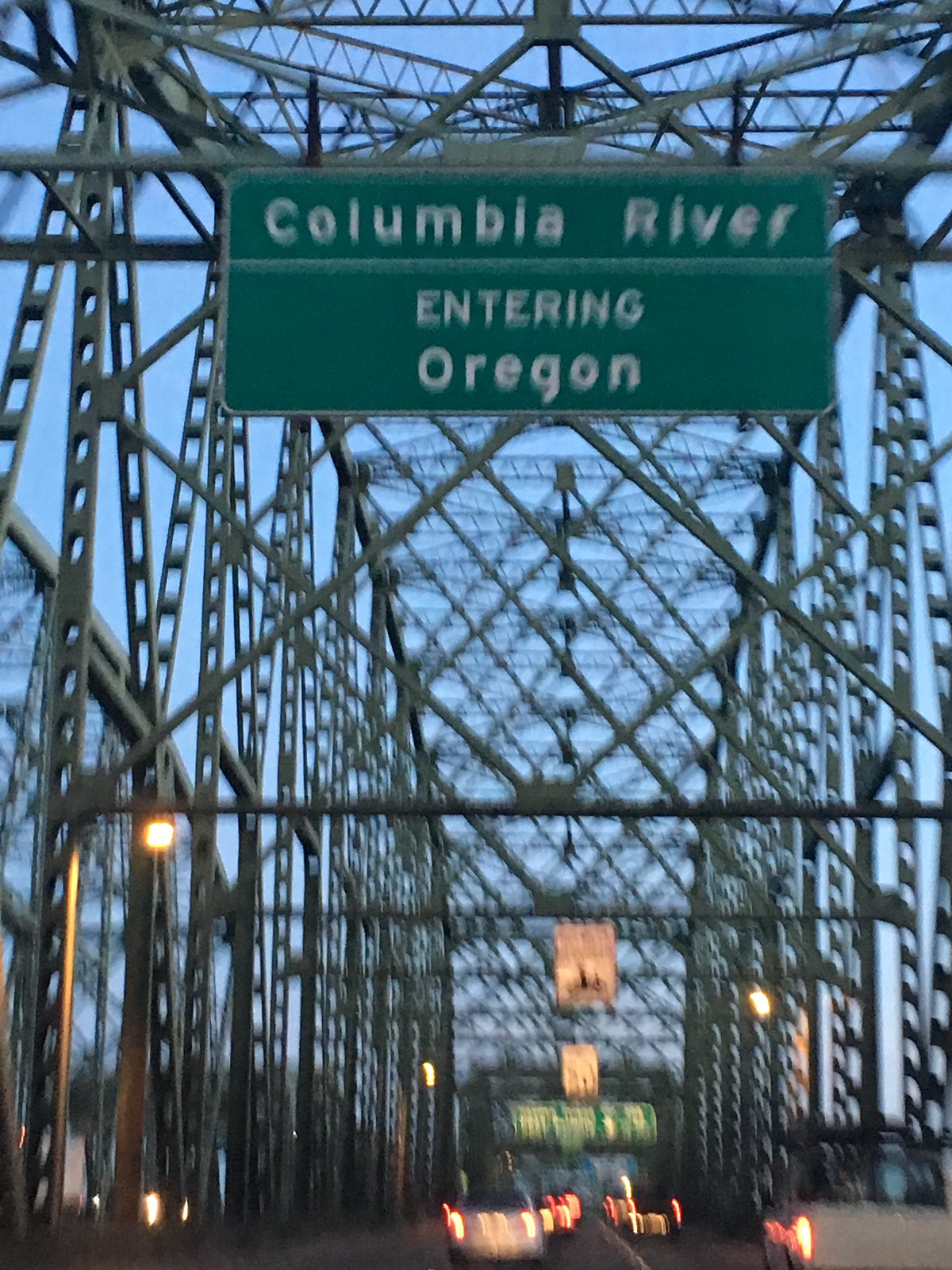The image captures a view from a car driving down a suspension bridge, leading toward Oregon, over the Columbia River. The perspective highlights the intricate metal framework of the bridge, forming a crosshatch, cage-like structure overhead. The scene appears to be either early morning or sunset, characterized by a vibrant blue sky tinged with hints of orange and purple near the horizon. The bridge has its own lighting, with the reflective glow of car headlights visible, further emphasizing the time of day. Prominently displayed is a green roadway sign with standard white lettering, reading "Columbia River" in bold, with "entering Oregon" in smaller capital letters beneath it. Additional signs, including white safety signs, hang from the bridge supports. The blurred nature of the photo suggests it was taken from a moving vehicle, accentuating the dynamic feel of the journey on this well-structured bridge.